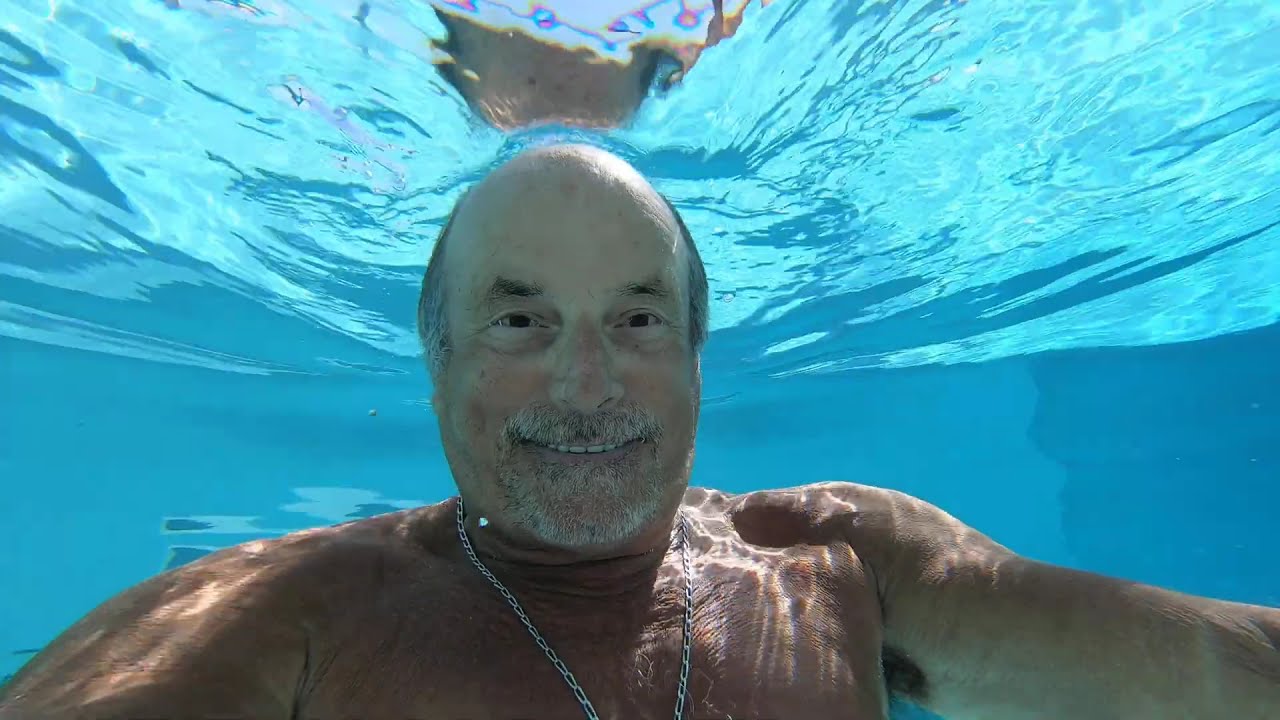In this underwater selfie taken in a crystal-clear aquamarine blue swimming pool, a smiling, middle-aged Caucasian man is positioned dead center. He has a bald top with some gray hair on the sides of his head, complemented by a salt-and-pepper beard and mustache around his lips and chin. He is shirtless and wears a silver chain necklace around his neck. The man, who appears to be in his fifties and has tanned skin, extends his arms in front of him to capture the selfie, making his hands not visible. His dark eyes and thin smile reveal a glimpse of his top teeth. Distortions and ripples in the water are visible, along with light reflections and a few bubbles around him, emphasizing the underwater ambiance. The backdrop consists of clear blue water, perhaps indicative of a pool setting, creating a serene and captivating scene.